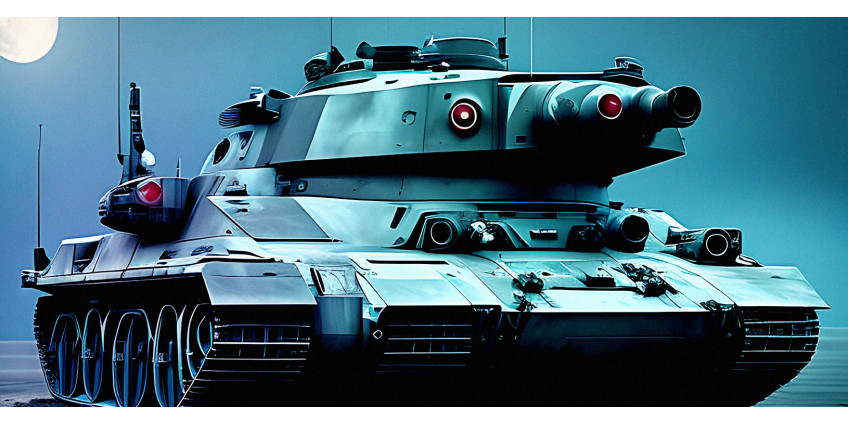The image is a detailed digital rendering of a futuristic tank set against a nighttime backdrop filled with varying shades of blue. The tank itself is predominantly blue with a shiny metallic finish, indicating its construction material. Its base and large treads, cropped slightly at the bottom, are dark blue to black, and the visible treads suggest a wide base with three tracks—two on the left and one on the right. The front of the tank features a prominent barrel, possibly equipped with a night vision scope and additional artillery with a heavy-duty scope. Red lights, reminiscent of headlights, adorn the tank’s various parts. Multiple antennas protrude from different points, emphasizing its advanced design. The background is minimal, dominated by a blue sky, with a glowing white moon positioned in the top left corner, enhancing the serene yet ominous atmosphere of the scene.